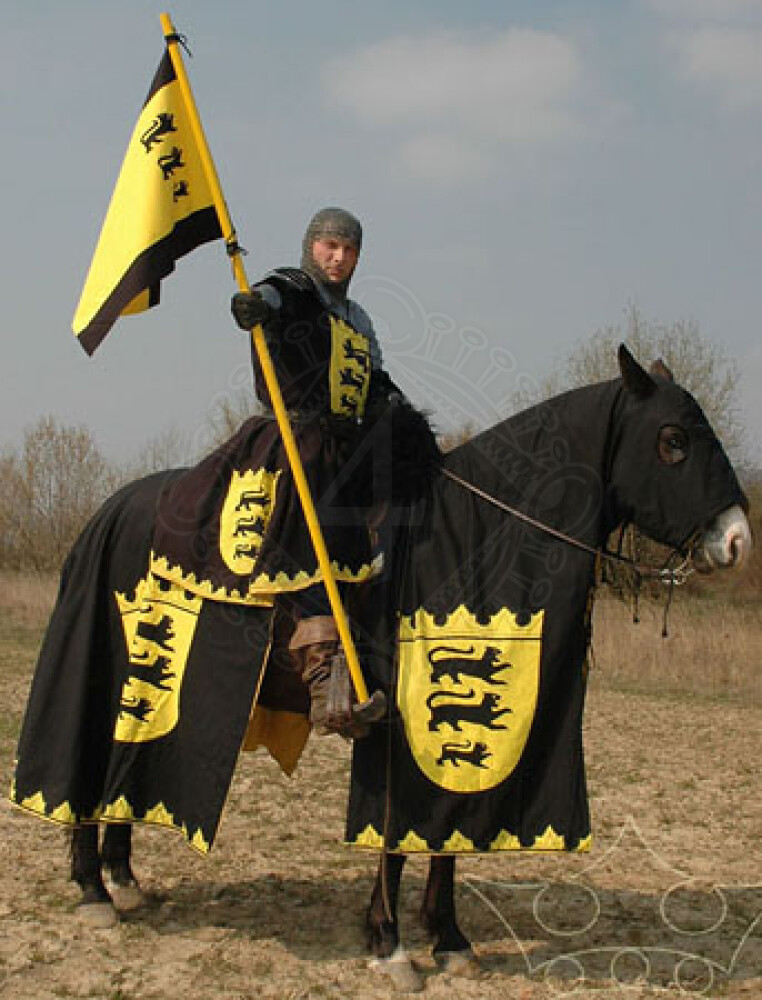This photograph captures a knight in full medieval regalia riding a horse, surrounded by an outdoor setting. The horse, standing upright and facing towards the right, is almost entirely draped in a black cover adorned with golden shields featuring repeated emblems of a panther or cougar. The knight mirrors this motif, wearing matching black and yellow attire with the same emblem displayed on both his chest and the side of his uniform. He holds a yellow and black flag, also emblazoned with the panther emblems, and his head is protected by a traditional chainmail coif. The background features a weedy, tree-dotted area under a gray, overcast sky, while the ground beneath the horse is a combination of brown dirt and sparse grass.